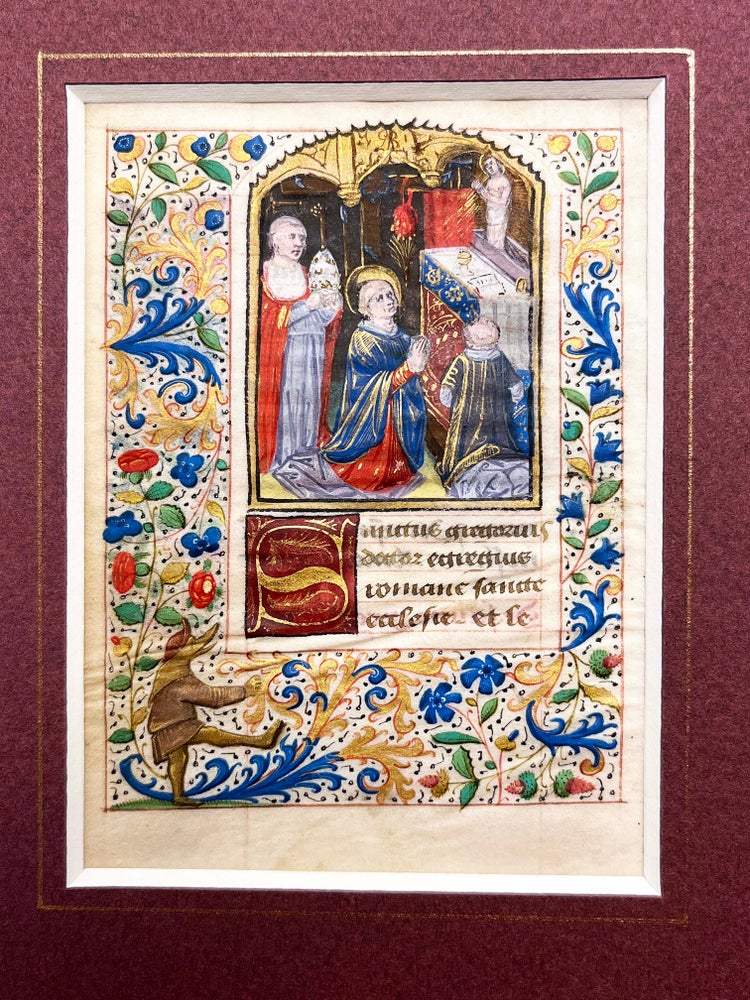This image is a framed, rectangular piece of artwork measuring approximately six inches high and four inches wide. The outer border is about three-quarters of an inch thick, adorned in a deep maroon color with light and dark blotches, resembling an ornate, possibly carpet-like texture. Inside this border, a thin gold strip encases an aged, yellowed paper that appears to feature biblical or religious content.

The main illustration on the paper is encircled with colorful images of leaves, flowers, and vines in shades of blue and gold. Within this decorative edge, in the lower left-hand corner, stands a humanoid figure with the head of an anthropomorphic animal. This figure, resembling a fox or a lizard with a long snout, wears a red hat, a brown outfit, and has gold and greenish legs. It poses dynamically, with its right leg kicked upwards and right hand extended outward.

Central to the artwork is a religious scene possibly depicting Apostles. One figure, dressed in blue robes with red details, kneels in prayer before a white altar covered with a cloth. Atop the altar, a smaller figure, perhaps representing Jesus Christ, is also praying, surrounded by golden lines or a halo. Nearby, another figure in a red robe stands, while other figures with golden crowns and robes are positioned around the scene. The figures' faces are light-colored, but lack fine detail.

Below this central vignette is a red square housing a large golden "S". To the right, there appears to be a section of gold print in a foreign language, likely Latin, set against a white background. The detailed patterns of the leaves and flowers, combined with the spiritual imagery, suggest this piece might be an excerpt from a religious scripture, carefully framed as a piece of historical and artistic significance.